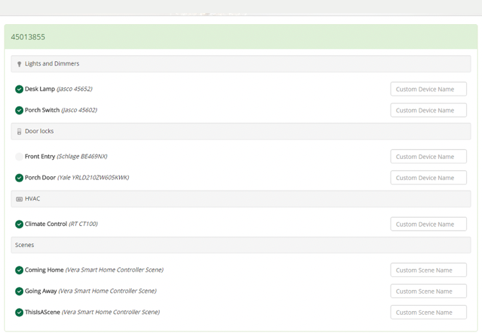The image is a screenshot from a home automation system interface, predominantly displaying a gray and white color scheme with various lines and texts. The topmost line is gray without any writing. Below it, there is a green line with the text "45013855" on the left side. Following this, a gray line labeled "Lights and dimmers" appears, accompanied by a small light bulb icon on its left. Subsequent lines alternate between white and gray backgrounds. 

- First white line: Checked with a green circle featuring a checkmark, labeled "Desk lamp."
- Next white line: Also checked with a green circle and checkmark, labeled "Porch switch."
- Following gray line: Labeled "Door locks."
- Next white line: Labeled "Front entry."
- Next white line: Checked with a green circle and checkmark, labeled "Porch door."
- Following gray line: Labeled "HVAC."
- Next white line: Checked with a green circle and checkmark, labeled "Climate control."
- Next gray line: Labeled "Scenes."
- Following three white lines: Each checked with a green circle and checkmark, labeled "Coming home," "Going away," and "This is a scene."

The interface seems to display various settings and statuses of connected home devices, indicating which ones are active or checked.